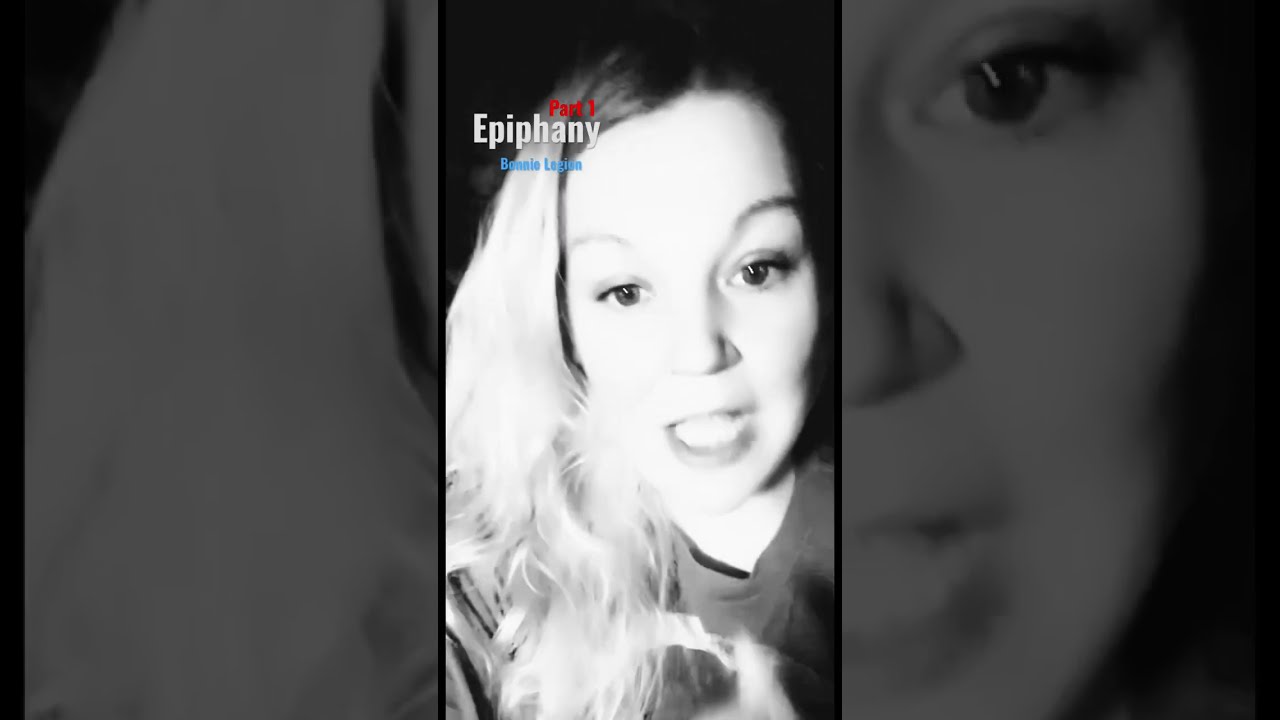The image is a vertically-oriented, high-definition black-and-white photograph, divided into three segments by vertical lines. In the center segment, there's a well-lit close-up of a woman's face. Her hair, which is dark on the top due to shadow, is parted slightly right of center and cascades down along the right side of her face, in front of her shoulder, and partially across her chest. She has brown eyes with raised eyelids, and her mouth is open, revealing her teeth, as if she is in mid-conversation. The woman is wearing a gray-colored shirt against a stark black background. The left and right segments are heavily tinted, zoomed-in portions of the central image. The left segment focuses on a close-up of her hair at the side of her face, while the right segment zooms in on her right eye and part of her nose. Text in the upper left corner of the central segment reads "Part 3" in red, "Epiphany" in white, and "Bonnie Legion" in blue.